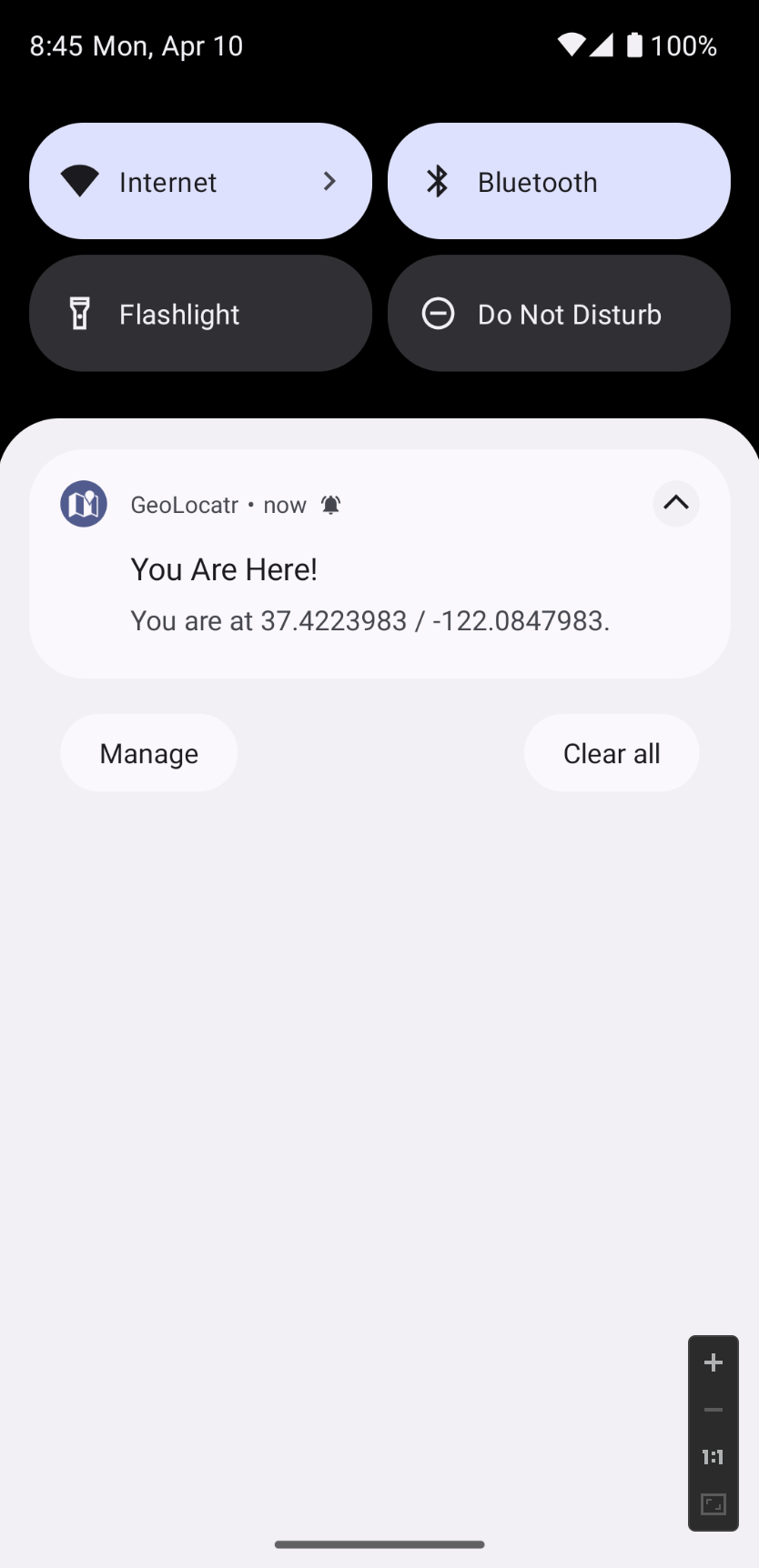This image, apparently captured from a smartphone screen, showcases a detailed view of the device's status and notification panel. The top-left corner displays the date and time as 8:45 AM on Monday, April 10th. Meanwhile, the top-right corner indicates a fully charged battery at 100%, along with strong Wi-Fi and cellular signals. Beneath these icons, tabs show that the Internet and Bluetooth functions are enabled. Below these, other quick-access buttons for flashlight and Do Not Disturb mode are visible. At the bottom section of the screen, there is an active Geolocator feature, pinpointing the user's current coordinates: latitude 37.4223983 and longitude -122.0847983, with an option to manage or clear notifications. The overall signal strength appears robust, indicating optimal connectivity.